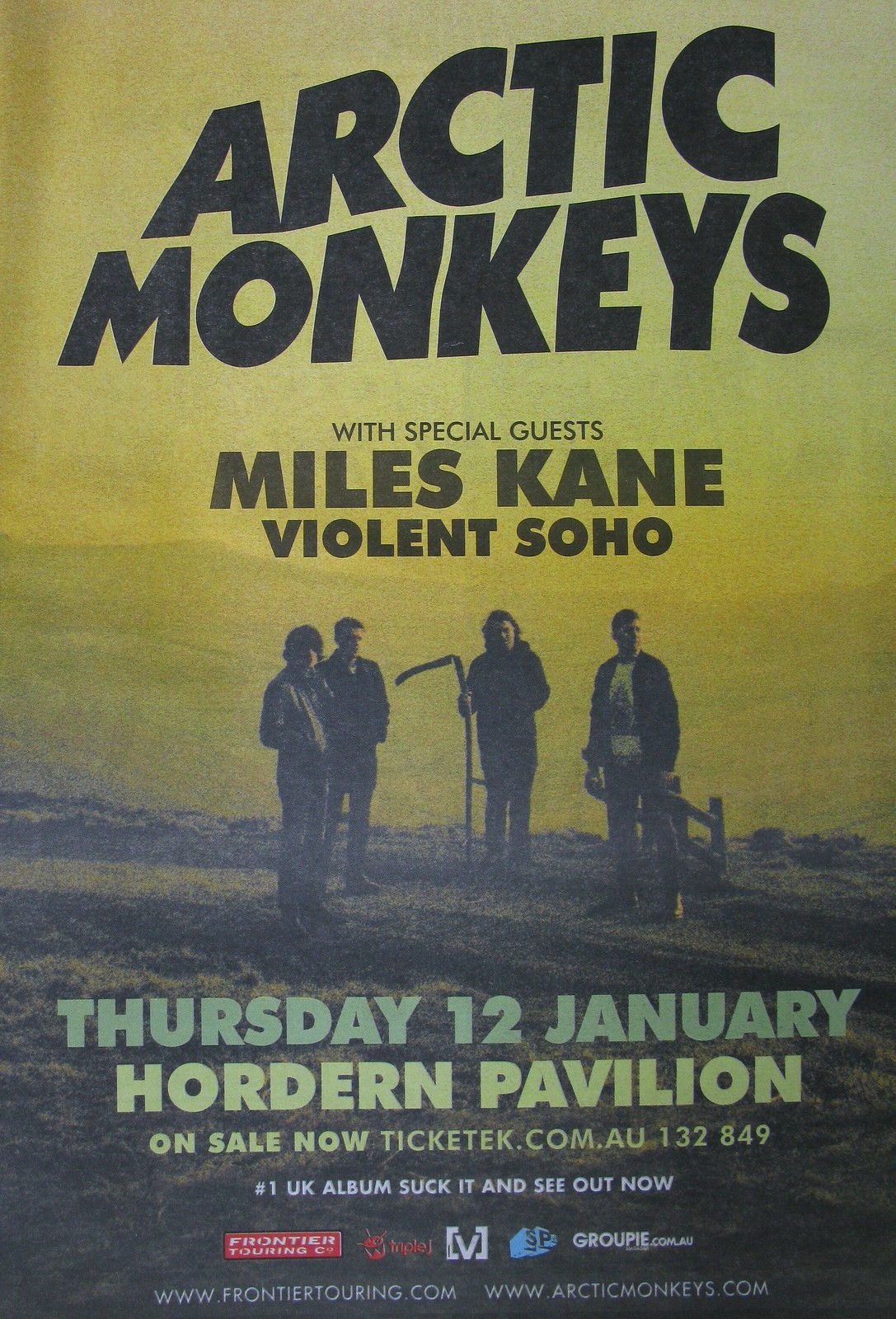This concert poster features the Arctic Monkeys prominently at the top, with special guests Miles Kane and Violent Soho. The background image showcases the four band members standing on a cliff with mountains behind them, looking in different directions, and one of them holding a scythe. The event details below the image read: "Thursday, 12 January, Hordern Pavilion." Tickets are available at ticketek.com.au with the contact number 132 849. In smaller font, it highlights the band's UK number one album "Suck It and See," which is out now. Additional sponsor information and websites for the Arctic Monkeys and Frontier Touring are also listed, including frontiertouring.com and arcticmonkeys.com.